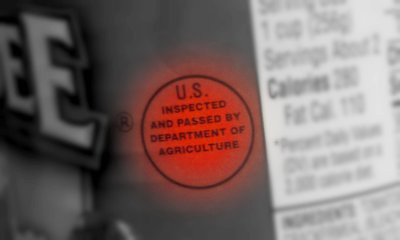The image depicts a close-up, black-and-white photo of a product package with a crop layout, focusing centrally on a distinct red highlight. Prominently featured in the red section is a black circle containing the label "U.S. inspected and passed by Department of Agriculture." On the left side of the image, the visible part of the product's name reveals two capital E's, though the full name is obscured. The bottom-left corner shows a small white section. To the right, the package's nutritional information is displayed, detailing that one cup equals 256 grams, with approximately two servings per package. Each serving contains around 260 calories, with 110 of those being fat calories. Although the ingredients are mentioned, the text is too small to read. The standout red highlight underscores the fact that the product has been inspected and approved by the Department of Agriculture.